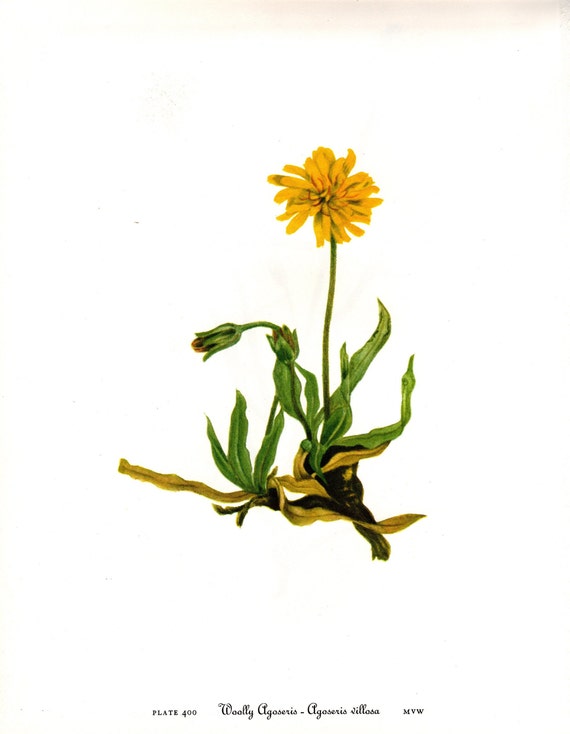This detailed artist's rendering depicts a vibrant yellow flower, identified as "Woolly Agoseris" (Agoseris villosa). The flower features high-volume petals arranged in a circular fashion around the bud, accented with red shoots at the center. A long green stem extends downward, where it meets additional elements: one stem bears an unopened bud that curls gracefully, and other stems and leaves, varying from green to brown, extend from the base. The illustration is set against a plain, white background with a slightly dirty texture near the top, with no indication of the environment's location. At the bottom left, the text reads "Plate 400, Woolly Agoseris - Agoseris villosa, MBW." Sparse green and brown leaves, resembling slender spigots of grass, can be seen around the base, suggesting minimal rooting into the soil.